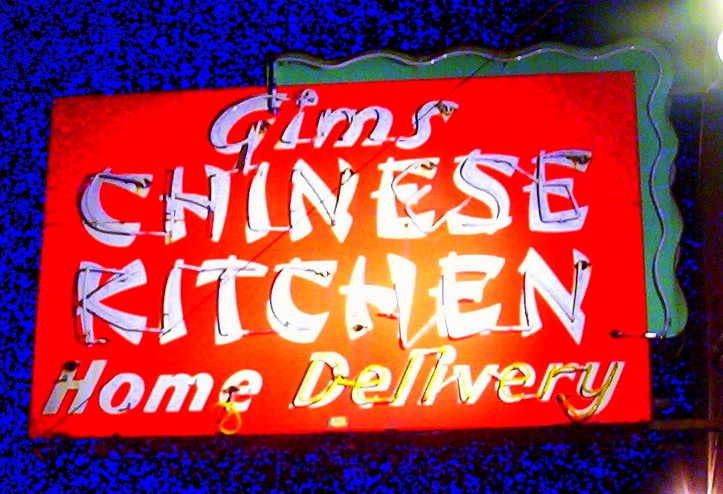The image depicts a non-illuminated, vintage red sign with lettering. The sign, which is likely for a Chinese food establishment, prominently features the text "GIMS Chinese Kitchen Home Delivery." The words "GIMS" and "Home Delivery" are in a regular font, while "Chinese Kitchen" appears in a style reminiscent of Chinese calligraphy. The text is predominantly light blue, but certain areas appear yellowish, possibly due to a spotlight effect.

The sign rests on a blue carpeted surface and an aqua ceramic object is visible in the top right corner. The background primarily consists of blue with black dots and includes a distinctive wavy, green rectangle in one area. The photograph is in landscape orientation and the scene is executed in a realistic, photographic style, showcasing the vintage design of the sign complete with visible neon light bars inside the lettering.